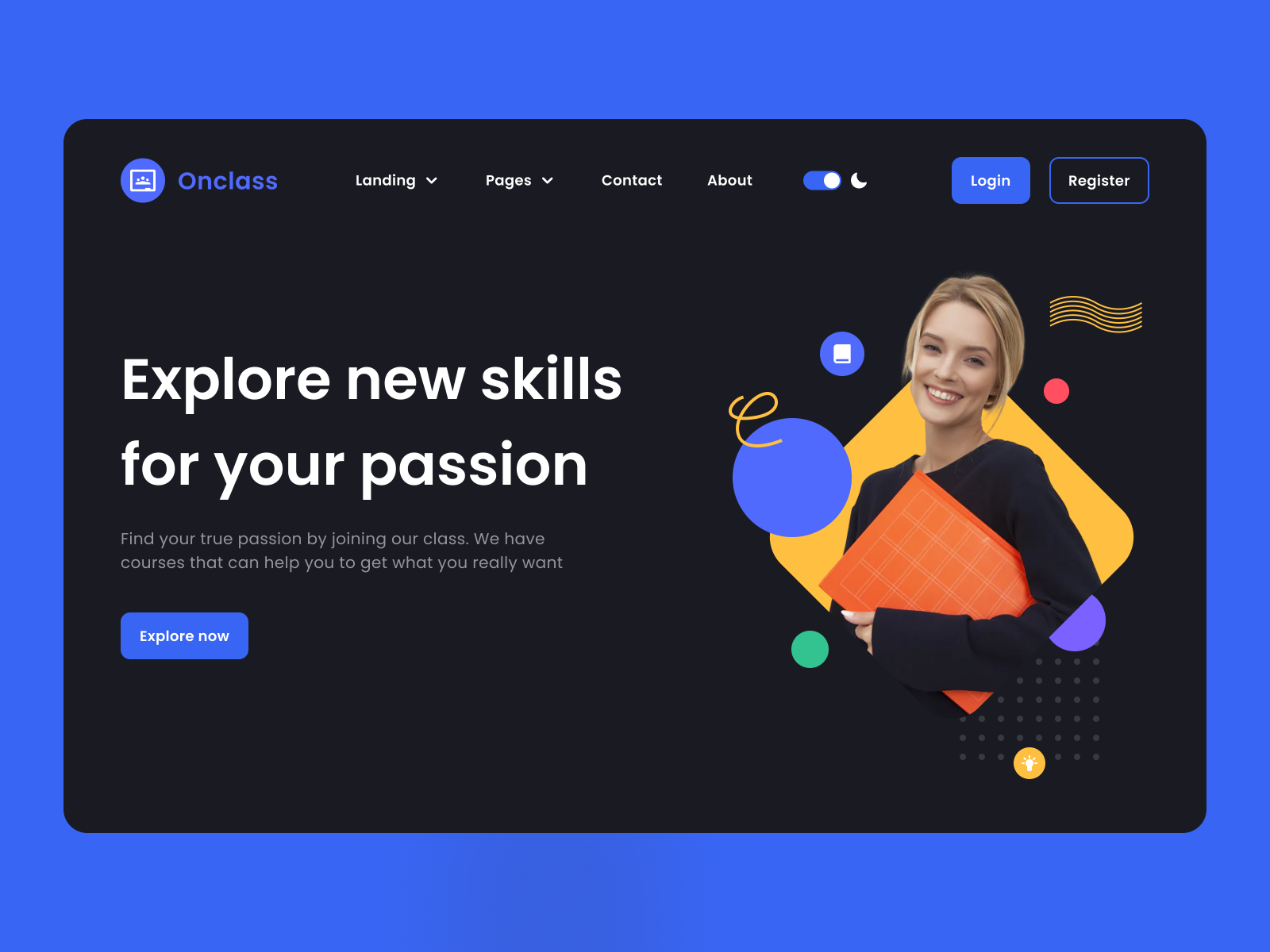In the background of the image, there's a rich blue color. Overlaying this is a prominent black rectangle positioned near the top. In the upper left corner of this black rectangle, there's a design element comprising a circle and a square, which share the same blue shade as the background. Inside the blue circle, there's a white square. Adjacent to this design, the phrase "On Class" is displayed in white.

Towards the right, there is a navigation bar with several tabs, including "Landing Pages," "Contact," and "About." Next to these tabs, there is a blue oval with a white left edge, which contains a white crescent shape. There are also two additional tabs: the first is solid blue and white, labeled "Log in," and the second has a blue outline with the word "Register" written in white.

On the left side of the image in white text, it reads: "Explore new skills for your passion. Find your true passion by joining our class. We have courses that can help you get what you really want." Below this text, there's a blue rectangular button with "Explore Now" written in white.

The image features a smiling woman, who appears to be white with blonde hair. She is wearing a long-sleeved black shirt and is holding a notebook with an orange and white stripe design. Behind her, there is a yellow diamond shape, and various multi-colored circles are scattered around her. These circles include colors like green, yellow, blue, purple, and red.